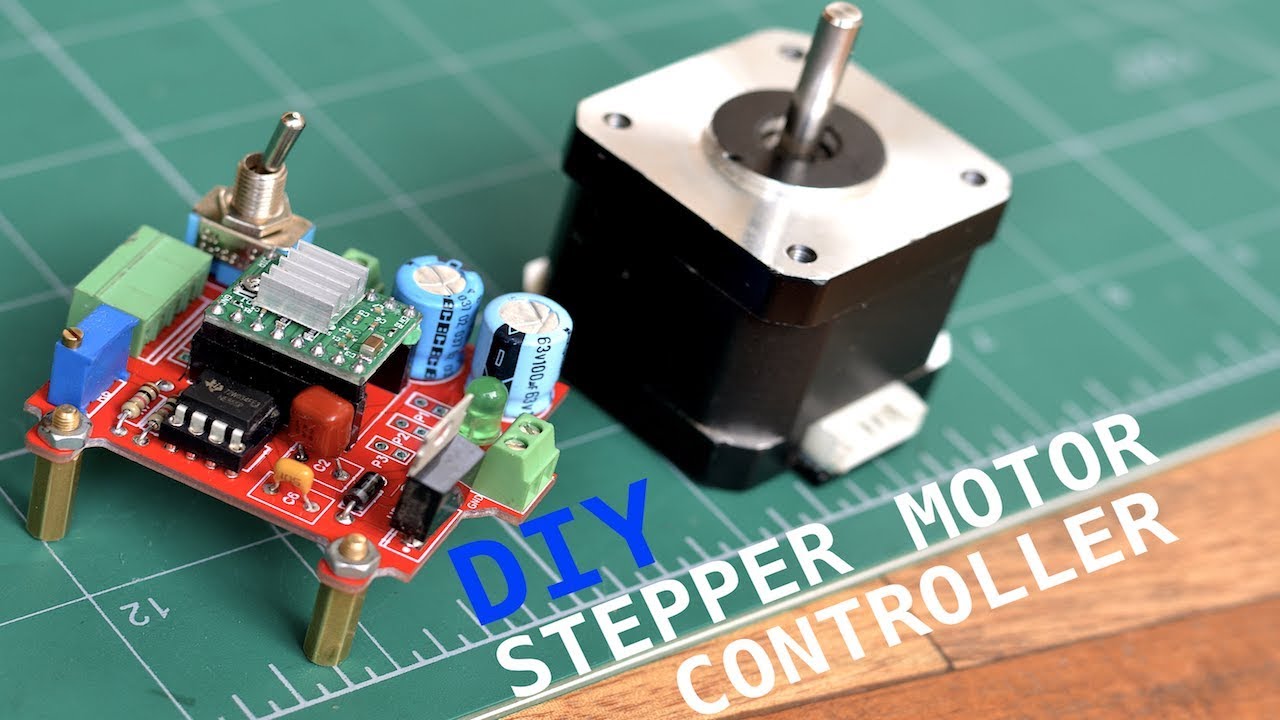The close-up image depicts a DIY stepper motor controller at the center, comprising two primary mechanical objects positioned on a green-bluish work surface that has the appearance of a calendar with a ruler edge. The first object is an exposed red printed circuit board (PCB) adorned with a variety of colorful components, including integrated circuits, resistors, capacitors, switches, bolts, LEDs, and what appear to be small batteries. The PCB is equipped with brass feet that elevate it slightly off the surface. Notably, a small switch is visible on one corner of the board. 

The second object, situated adjacent to the PCB, resembles a joystick or control lever encased within a sealed, black, metal square with a silver top, offering no insight into its internal workings. An inscription on the photograph clearly identifies this set-up as a "DIY Stepper Motor Controller." Both objects rest atop what appears to be an electrically safe plastic work surface suitable for electronic projects. This detailed display likely serves as an advertisement or instructional image for DIY enthusiasts.